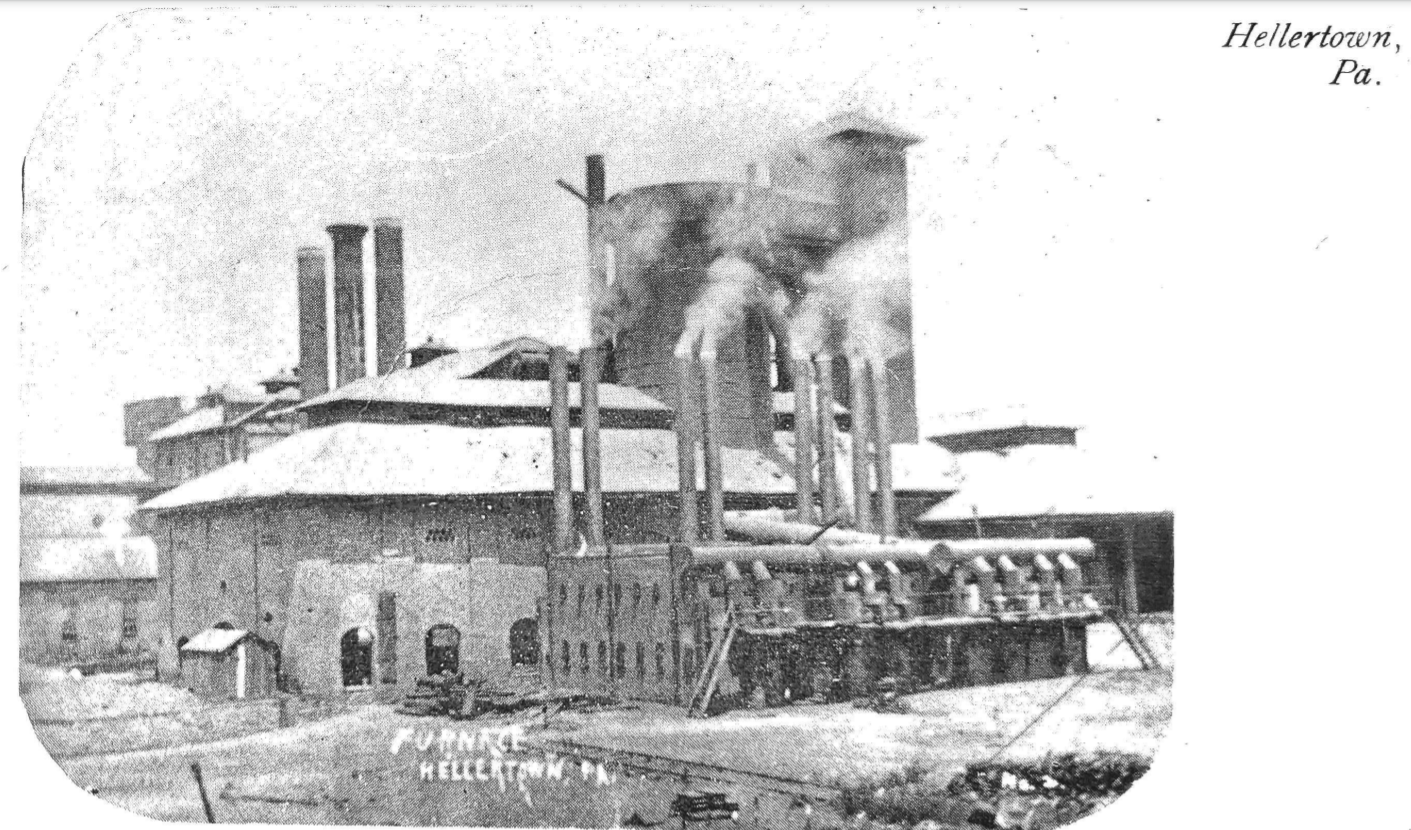This is an aged, black-and-white landscape photograph of an industrial site in Hellertown, Pennsylvania. The image is faded and shows signs of wear with slight curves at its corners. The main focal point is a large manufacturing building, likely a furnace, as indicated by the white text at the bottom which reads "Furnace, Hellertown, Pennsylvania." In the upper right corner, it also says "Hellertown, Pennsylvania" in black text over the image.

The factory complex is detailed with several prominent features: the central building is expansive, constructed of concrete, and marked by numerous oval-shaped entrances and windows. There are at least eight large smokestacks at the forefront emitting smoke, with three additional stacks visible behind. The building's exterior is adorned with various large pipes, possibly part of HVAC or generator systems. Behind the main structure, large brick buildings and two towering silos are also visible, suggesting a substantial industrial operation. Chain-link fences can be seen around the perimeter, adding to the industrial atmosphere. The entire scene, set against a snowy landscape, evokes a sense of a bygone era of manufacturing.